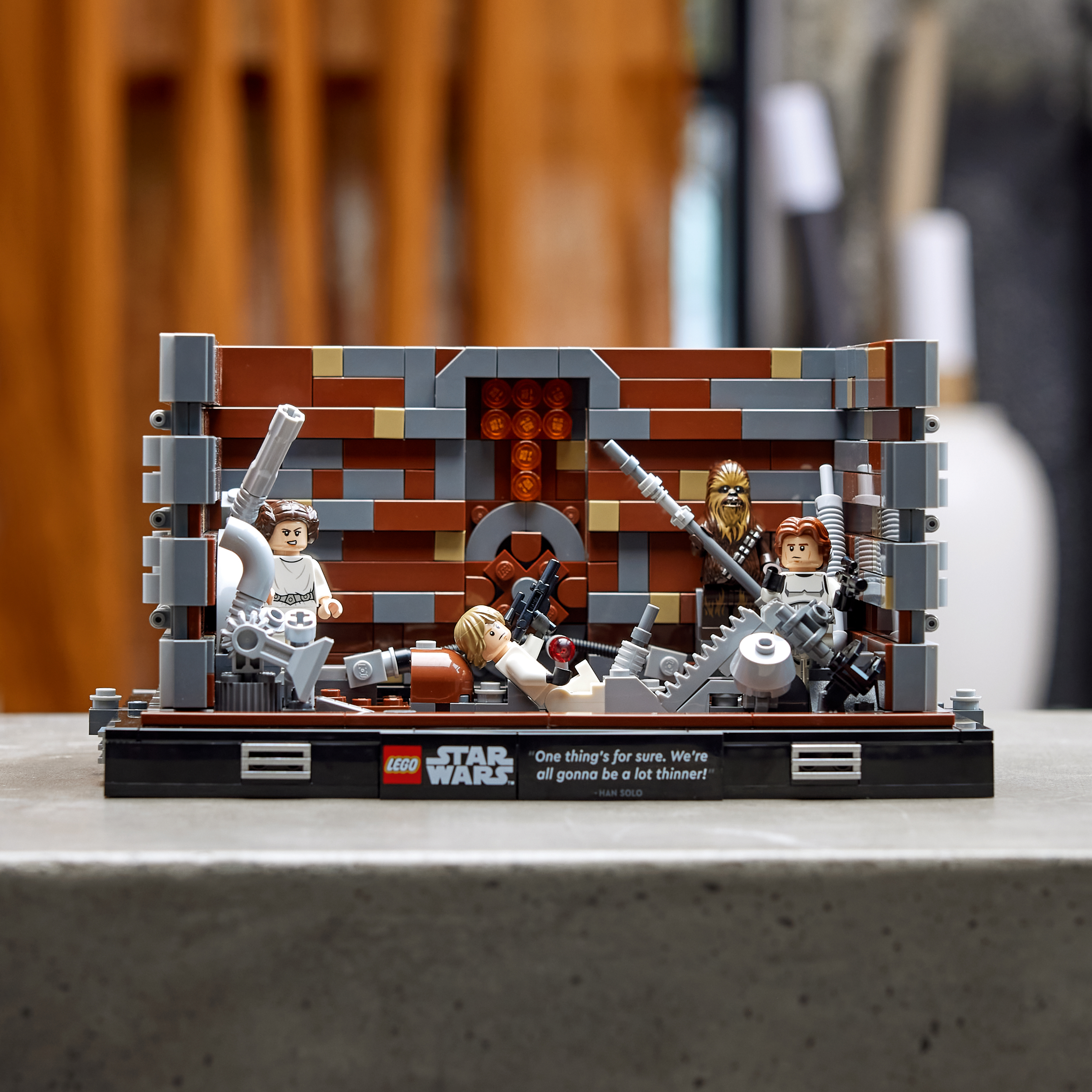The image shows a sharply focused CGI representation of a meticulously assembled LEGO Star Wars set placed on a marble table. The background is intentionally blurred to emphasize the figures in the foreground. Prominently featured are LEGO versions of Chewbacca, Princess Leia, and Luke Skywalker, poised as if preparing for a battle, with some characters visibly carrying weapons. The text overlay reads, "One thing's for sure, we're all gonna be a lot thinner." The color palette of the LEGO set is a rich mixture of colors including orange, gray, silver, dark red, gold, white, brown, and black, enhancing the vivid and dynamic scene. The setting and styling suggest an indoor environment conducive to the detailed display of the LEGO figures.